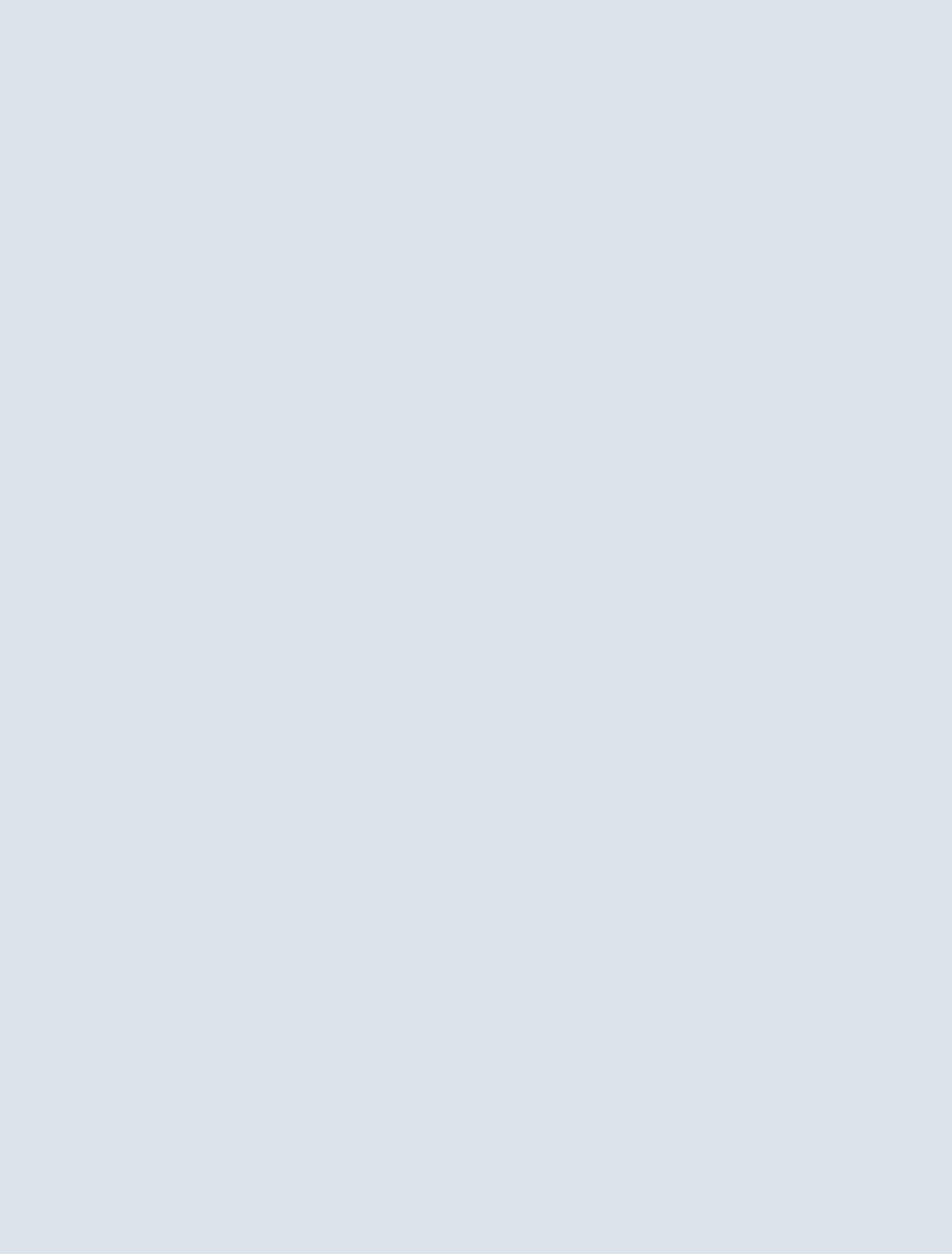A rectangular image featuring a flawless expanse of light blue dominates the visual field. The proportions of the rectangle are such that the top and bottom edges are shorter, while the left and right sides extend longer, reinforcing its rectangular shape. The blue hue is consistently applied across the entire image, showing no variation or gradient. This particular shade of blue is reminiscent of a lightly clouded sky on a coastal day, where the blue sky peeks through a thin veil of mist or fog. The blue is neither a vivid baby blue nor a stark brightness but rather a serene, airy light blue interspersed with subtle hints of white. The image is devoid of any forms, figures, or additional features, presenting a pure, uninterrupted wash of tranquil color.